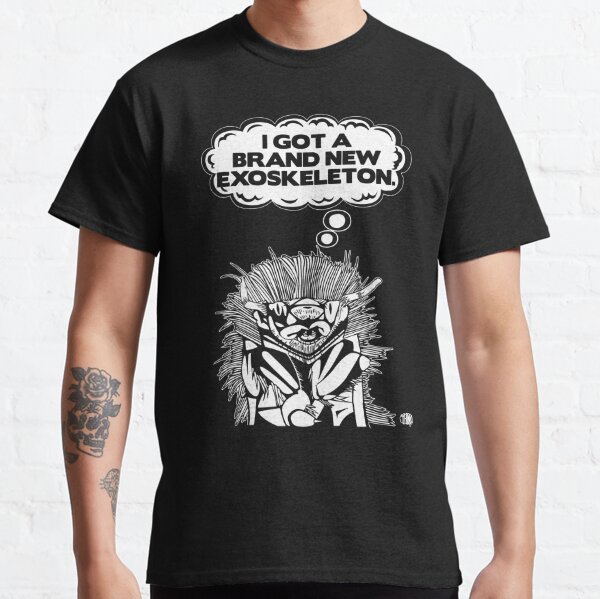This is an image of a young Caucasian man wearing a black short-sleeved cotton t-shirt, depicted in a portrait layout. The photograph primarily focuses on the t-shirt, which bears a distinctive graphic design in the center. The design features a black and white creature with a thought bubble that reads, "I got a brand new exoskeleton." The man's face is not visible in the image, but you can see his neck and his tattooed arms. The tattoo on his right forearm features roses, along with other indiscernible elements. He is also wearing black pants. The overall composition highlights the graphic design of the t-shirt and the man's arm tattoos against a plain backdrop.